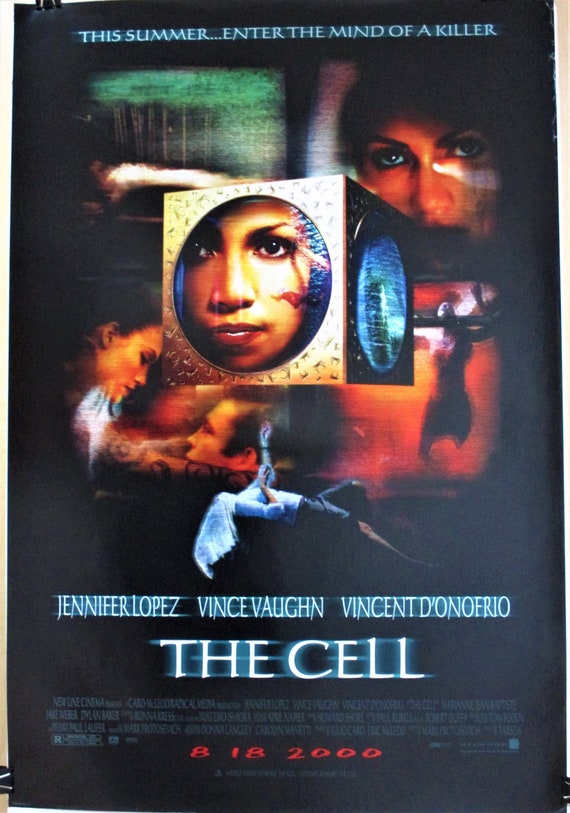The image is a dark and ominous movie poster with a charcoal gray and dark brown background. At the top, in bold white lettering, it reads, "This summer enter the mind of a killer." Below, at the bottom, also in white, are the names Jennifer Lopez, Vince Vaughn, and Vincent D'Onofrio, followed by the blurred title of the movie, "The Cell." A red, partially illegible date — likely August 18, 2000 — is on the poster along with tiny white credits. Dominating the center is a gold, square picture frame resembling a portal, through which a face peers intensely. The image within the frame consists of a dark-haired woman’s face, partially obscured and blurred, evoking a sense of eerie mystery. Around this are varying shades of orange, rust brown, green, and a touch of ice blue, suggesting swirling clouds that enhance the surreal and foreboding atmosphere of the poster.